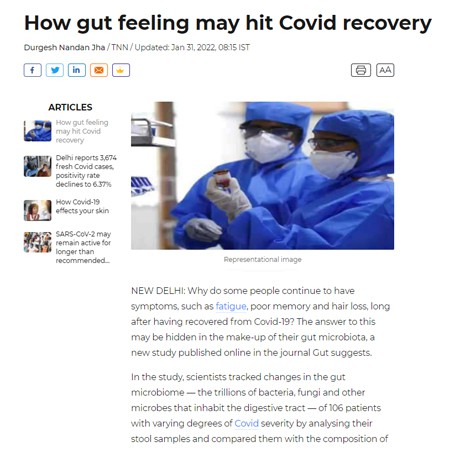Screenshot Description: Indian Online News Article Discussing Long COVID and Gut Health

The image is a slightly out-of-focus screenshot from an Indian online news website. Dominating the right side of the webpage is a large, representational photograph of two healthcare or lab workers. They are clad in blue protective coveralls, complete with matching hoods, N95 respirator masks, goggles, and latex gloves. One worker, presumed female, holds a sample jar in her left hand, while standing in front of a lab shelf, further suggesting a laboratory setting.

The article's headline, prominently displayed, reads: "How Gut Feeling May Hit COVID Recovery." The piece is authored by Durgesh Nandan Jha, with the initials 'TNN' indicating his affiliation. It was last updated on January 31, 2022, at 08:15 IST (Indian Standard Time).

Directly beneath the headline is a horizontal row of social media icons, including Facebook, Twitter, and Instagram, along with a few unrecognized logos. Along the left side of the page, there's a vertical column of article thumbnails labeled "Articles," allowing readers to navigate between different stories. Currently highlighted is the featured article titled, "How Gut Feeling May Hit COVID Recovery."

Other clickable article titles include:
1. "Delhi Reports [Number] Fresh COVID Cases; Positivity Rate Declines to 6.37%"
2. "How COVID-19 Affects Your Skin"
3. "SARS-CoV-2 May Remain Active for Longer Than Recommended"

The main article begins by posing the question: "Why do some people continue to have symptoms such as fatigue, poor memory, and hair loss long after having recovered from COVID-19?" It suggests that the answer may lie in the composition of their gut microbiota, according to a new study published in the journal 'Gut.' The term "fatigue" is hyperlinked, allowing readers to access more information. The subsequent paragraph discusses the study in detail, noting that scientists tracked changes in the gut microbiome of 106 patients with varying COVID-19 severity by analyzing stool samples and comparing them with healthy subjects. The word 'COVID' is also a clickable hyperlink.

The rest of the article's content is cropped off in the screenshot.